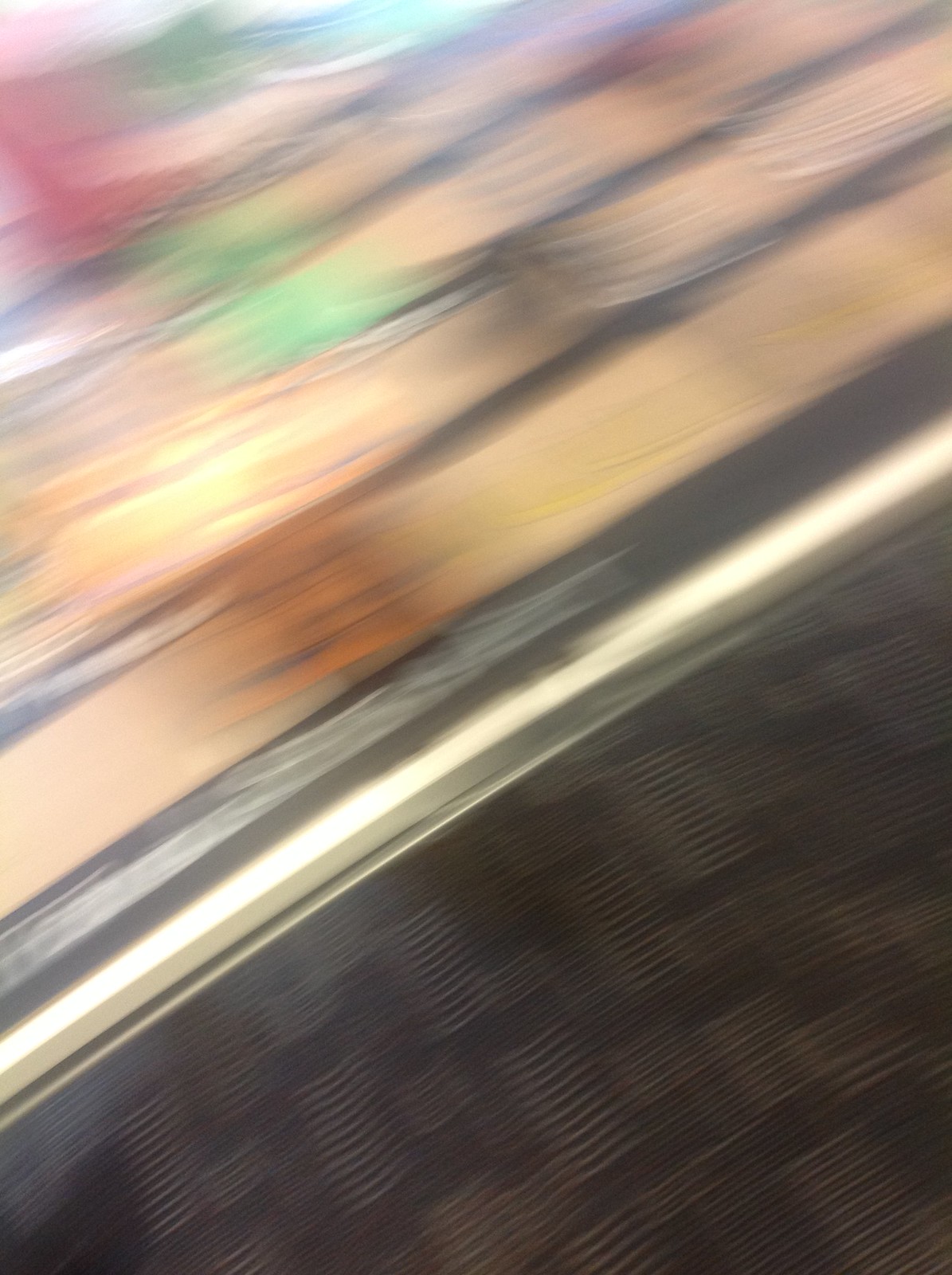Blurry image of a detailed wicker basket: The basket appears to have a dark brown base, with a silver band featuring a sharp, pointed edge positioned above it. Above the silver band is a section wrapped in black paper or a similar material. The main body of the basket consists of five layers of intricately woven wood. The bottom two layers contain yellow accents. The subsequent two layers display green tones, followed by red at the top and additional green and blue elements.